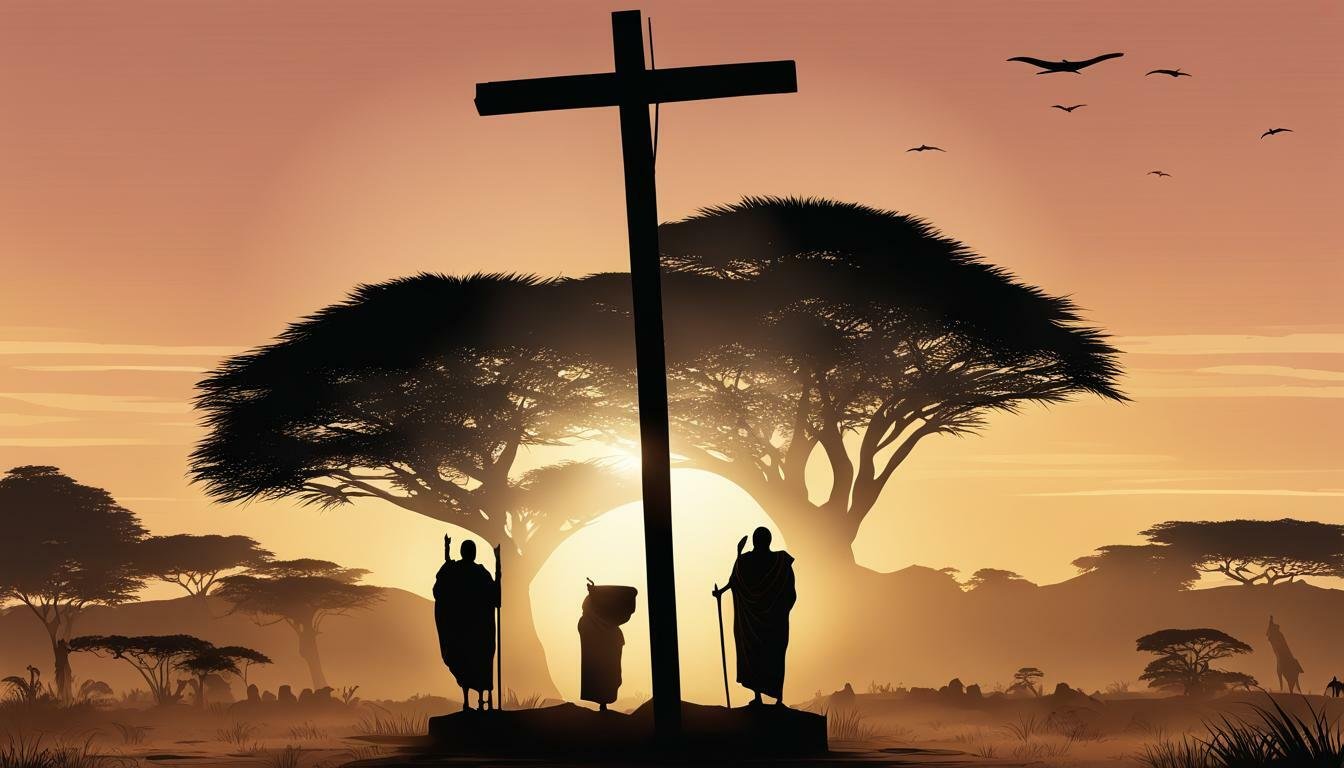The rectangular image is a detailed silhouette drawing centered around a tall, prominent wooden cross, which extends vertically to the top of the frame. Flanking the cross are two robed figures, each holding staffs, and positioned on either side atop a rocky pedestal. The figure on the left holds a long staff in his left hand and has his right hand raised, while the figure on the right grips a shorter staff. Additionally, there seems to be another small creature-like silhouette with a disproportionately large head nearby.

In the background, a forest scene unfolds with trees framing the cross—two significant trees on either side and more trees to the left and right. The sun is setting, casting a golden light through a circular gap between the trees directly behind the cross, imparting a serene, almost sacred ambiance to the scene. The sky transitions from pink to orange hues, adorned with light, wispy white clouds stretching across the middle. In the upper right corner, the outlines of several birds are visible, flying high in the sky. The lower part of the image features tall grass peeking out from the right side, contributing to the natural, tranquil setting.